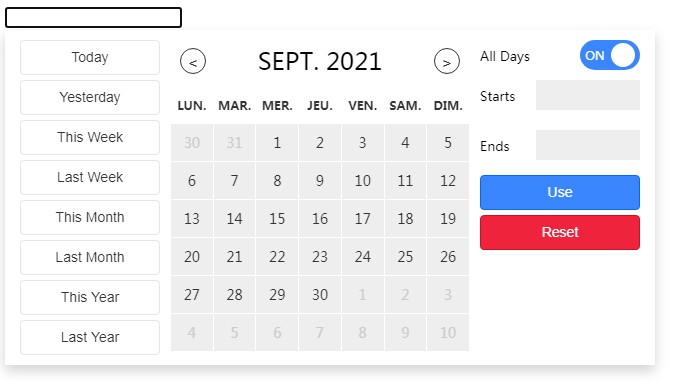This image depicts a detailed view of a digital calendar interface dated September 2021. On the left side, there is a vertical toolbar with a header bar outlined in black but containing no content. Below this header, the toolbar features a list of time frame options—Today, Yesterday, This Week, Last Week, This Month, Last Month, This Year, and Last Year.

The calendar itself is flanked by navigation arrows on either side, allowing the user to switch to the previous or next month. The days of the week are represented with abbreviations in French: Lun (Monday), Mar (Tuesday), Mer (Wednesday), Ju (Thursday), Ven (Friday), Sam (Saturday), and Dim (Sunday). The calendar grid begins with the 30th of August and extends to the 10th of October, with September occupying the central portion.

On the right side of the calendar, there is an "All Days" toggle switch, which is currently turned on and displayed in blue with a white circle. Adjacent to where the calendar starts and ends, there are gray boxes to demarcate these points. 

Beneath the calendar grid, there is a blue "Use" button and a red "Reset" button for user actions. The overall color scheme of the interface includes the blue "Use" button, the red "Reset" button, and the blue "All Days" toggle switch, with the rest of the interface following a grayscale theme.